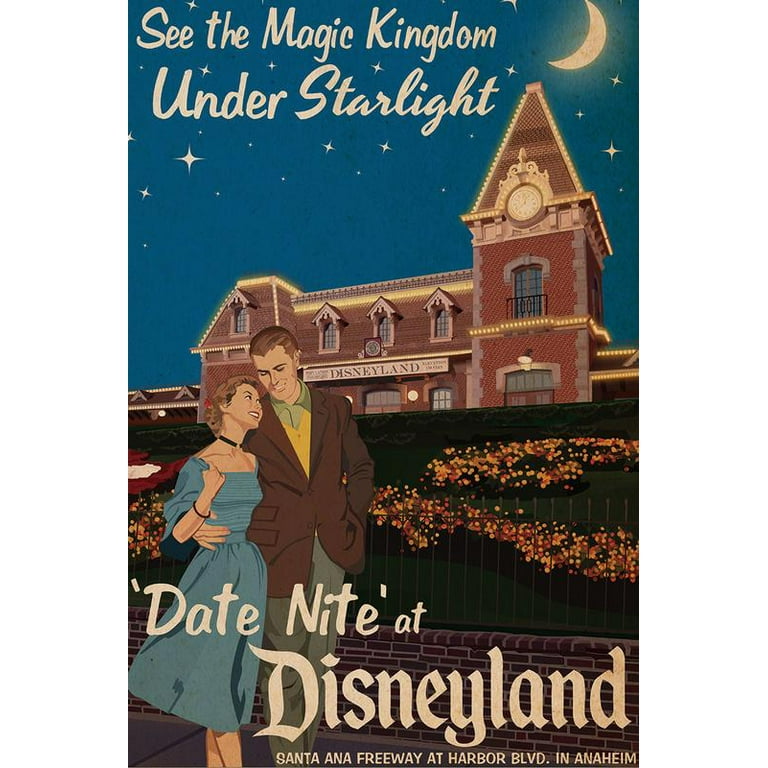This image, likely a vintage flyer or poster from anywhere between the 50s and the 80s, features a color painting of Disneyland at night. Central to the image is a large, charming brick building with a clock tower on the right side, illuminated by lights along its trim, and a prominent "Disneyland" sign on its facade. Above, a text in white reads, "See the Magic Kingdom Under Starlight," accompanied by a twinkling starry night sky and a crescent moon. In the foreground, a man in a green-collared shirt, yellow vest, brown jacket, and grey pants, walks alongside a woman dressed in a blue dress with a black choker. They stroll past a hill adorned with red, yellow, and white flowers. At the bottom, another text in white announces, "Date Night at Disneyland," with additional details noting the location: "Santa Ana Freeway at Harbor Boulevard in Anaheim."